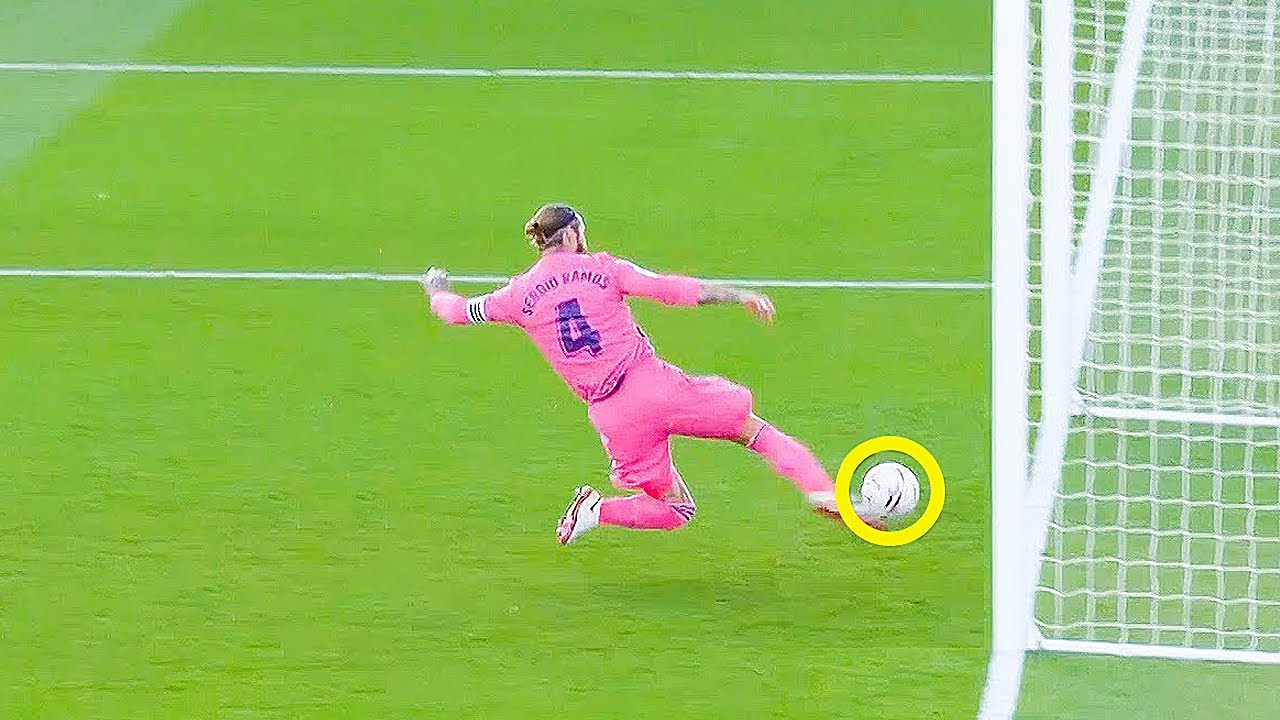The image captures an action-packed moment during a soccer match, featuring a player in a striking pink uniform. The central figure, identified as Sergio Bandez or possibly Sergio Ramos, is airborne mid-kick, his entire body in dynamic motion as he interacts with the ball, which is highlighted by a yellow circle, indicating a replay. Sergio, with a ponytail secured by a headband, also wears a white armband. The number four is visible on his back. The shot is tightly focused on him, showing a ten-foot radius around him with no other players or a goalkeeper in sight. The lush green grass and the presence of a soccer net suggest he might be either scoring a goal or performing a crucial defensive move. The clarity in the details like his pink socks, pink uniform, and white-pink shoes adds to the vibrant energy of the scene, making it a vivid depiction of a high-stakes moment in the game.